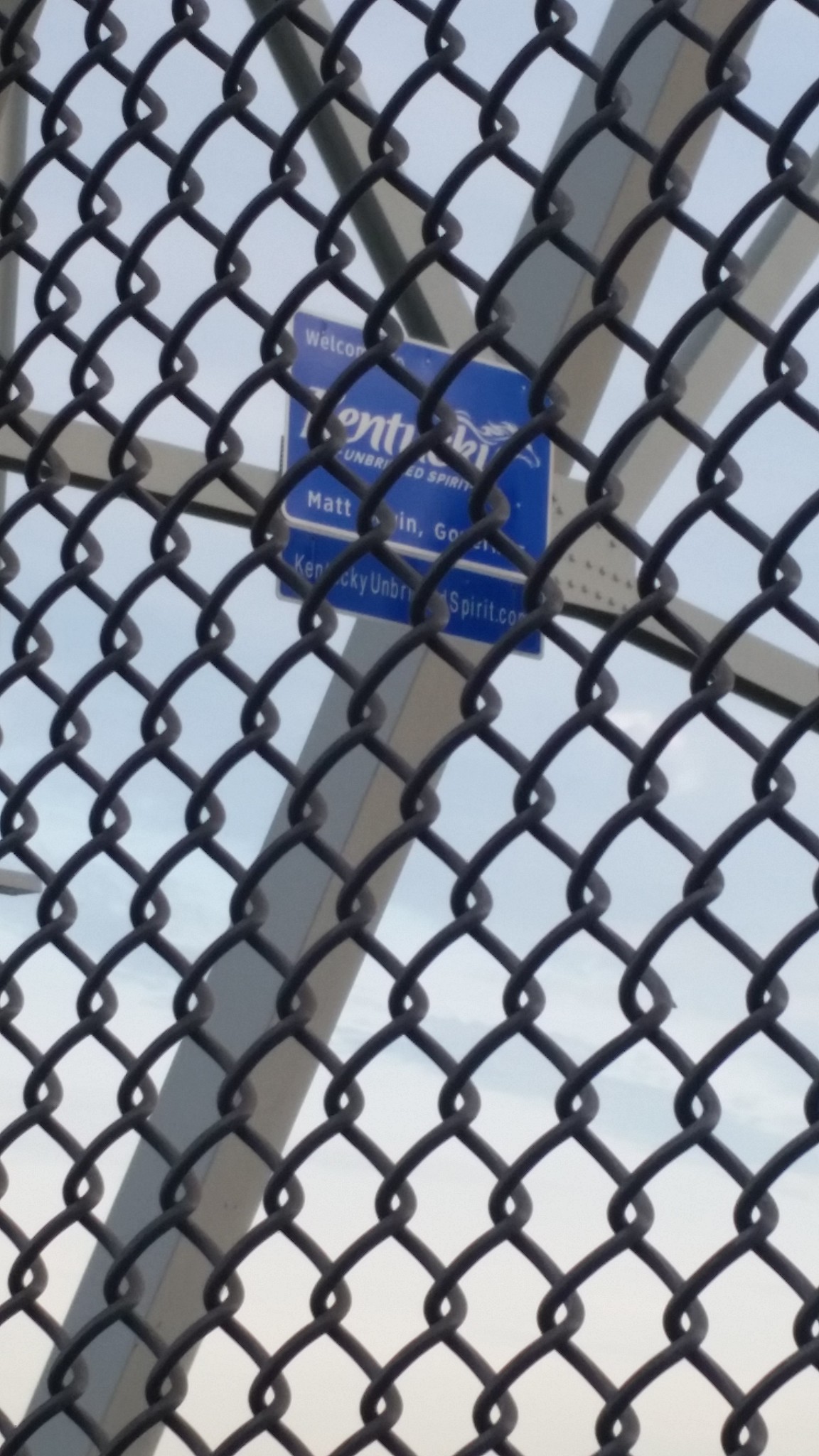In the photograph, there is a black chain link fence prominently featured in the foreground. Above the fence, a sturdy metal structure is visible. The structure includes a large metal bar extending diagonally from the lower left to the upper right. Intersecting this bar is a smaller, horizontal metal bar that spans from left to right. Additionally, two more metal bars radiate outward at 45-degree angles toward the top of the image, creating a symmetrical, geometric pattern.

Attached to the horizontal cross piece is a blue sign. The sign bears the word "Kentucky" in bold, white letters, and is clearly visible. Through one of the holes in the chain link fence, beneath the word "Kentucky," the word "Matt" can be discerned printed on the same blue sign. The careful arrangement of the metal bars and the strategic positioning of the sign provide a well-composed visual that draws attention to both the structural elements and the signage.